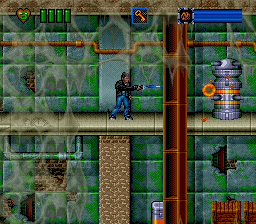This image is a detailed screenshot from what appears to be a 90s-style video game or a modern game designed to look retro. The image, although cropped and of modest quality, reveals a character dressed in blue pants and a black jacket who is crouched and seemingly shooting a gun. The background features green tiled walls with visible pipes and areas where tiles have fallen away to expose brick underneath, giving the impression of a dilapidated, multi-story underground environment.

At the upper left corner, there is a heart symbol with the number '3' inside it, accompanied by four rectangular green bars, likely representing the character's health and status. Positioned slightly to the right, there is a blue box with an orange key logo inside it. The upper right corner displays a long blue rectangular bar that could signify the character's stamina or energy.

On the right side of the scene, a metallic robot with an orange glowing part stands near a series of wooden boxes. The misty effect overlaying the entire image adds to the vintage atmosphere. This intricate composition captures various layered elements that contribute to the game's challenging environment and nostalgic visual style.